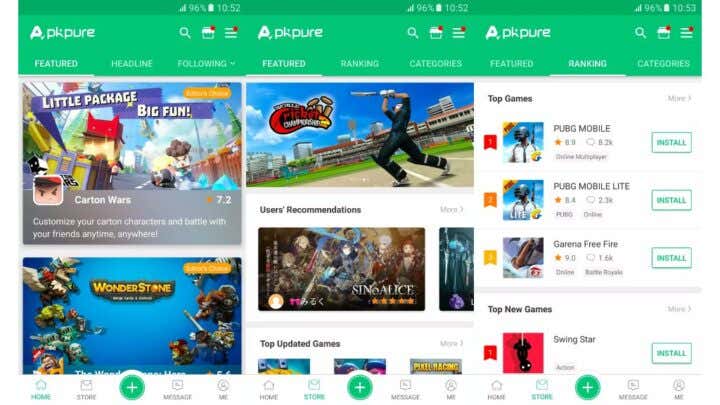The image displays a smartphone screen showcasing the APK Pure app interface. At the top, several tabs titled "Featured," "Headline," "Following," "Featured Ranking," and "Categories" are aligned next to each other. The battery icon indicates a charge level of 90%, and the time reads 10:52 AM.

Beneath the tabs, there are several promotional images for different mobile games and applications. One prominent image promotes "Little Big Fun," featuring the game "Cartoon Wars" with a caption that reads, "Customize your cartoon characters and battle with your friends anytime, anywhere." Adjacent to it, another image features "Wonderstone," but no further information or directions are visible.

At the bottom of the screen, a navigation bar displays icons for "Home," "Store," "Add," and "Message." Just above this navigation bar, a section showcases user recommendations and popular game titles, including "Sinalis," "PUBG Mobile," "PUBG Mobile Lite," and "Garena Free Fire," each accompanied by buttons to install them. The interface is designed to provide a user-friendly experience, with easy access to a variety of gaming and app options.